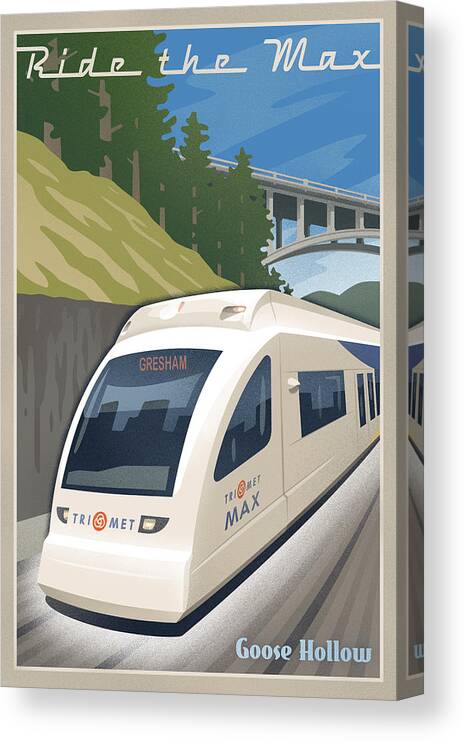The image is a detailed artist's conception of a sleek, high-speed Max Light Rail train, depicted on what appears to be a vintage canvas travel poster. The high-speed train, characterized by its aerodynamic, sloped front, is predominantly white with a large, square window at the front that displays "Gresham" in yellow, indicating its destination. The front of the train also features the TriMet logo, with "TriMet Max" marked below the headlights.

The train is shown traveling along a track toward the lower left corner of the image, with a cement trestle bridge overhead. The landscape includes a green hill adorned with pine trees along the left, and a long tall cement wall runs parallel to the track, providing stability against the hillside. Near the bottom right corner of the picture, the name "Goose Hollow" is indicated, possibly referring to the artist or the location. The top of the poster prominently displays the phrase "Ride the Max," inviting viewers to take part in this modern transit experience.